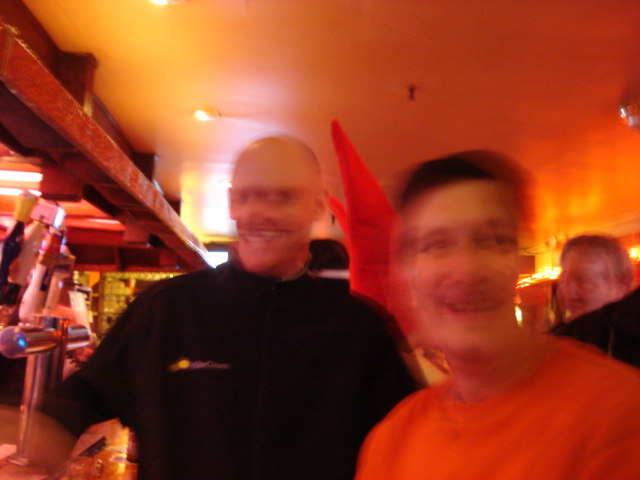In this somewhat blurry photo likely taken at a bar, three men are captured in motion. The man in the forefront, with short hair and possibly a mustache, is wearing a red shirt and smiling at the camera. To his right, but on the left side of the image, stands a taller man with a bald head donning a black shirt. Slightly behind them, on the right side of the photograph, another individual, probably male, is partially visible in the background. The blur suggests either the subjects were moving, or the camera was in motion during the shot. The warm atmosphere and background details hint that the setting is a lively bar.